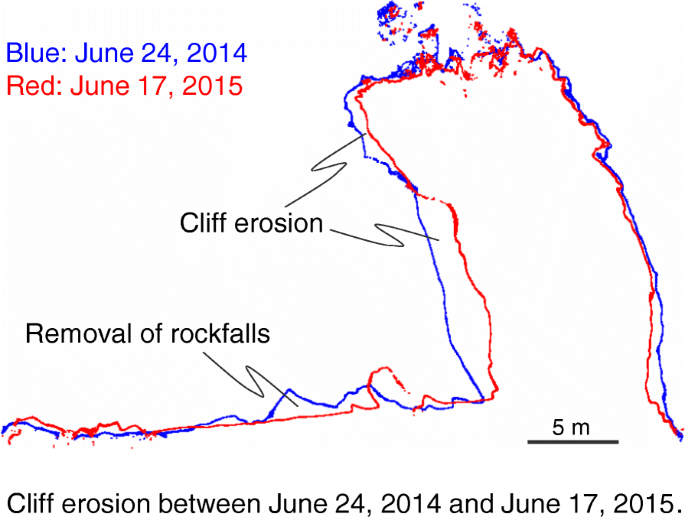This detailed digital chart features a white background with no definitive border, containing intersecting red and blue lines that represent changes over time. The blue line, labeled "June 24th, 2014," traces a path starting from the lower left, moving to the center, then ascending and dipping towards the lower right. Similarly, the red line, marked "June 17th, 2015," follows a comparative trajectory, highlighting cliff erosion and rock fall removal between these two dates. The graph visually depicts the extent of cliff erosion, showing where the cliffs eroded from the initial position indicated by the blue line to the later state marked by the red line.